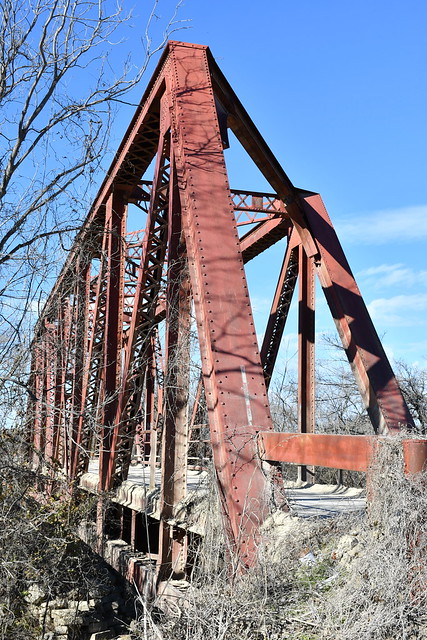This photograph, taken in portrait orientation, captures a rusty orange-brown metal bridge, possibly a steel suspension bridge, that looks aged and neglected. The structure is distinguished by its numerous intersecting beams forming triangles and upright columns attached to rocky supports. The bridge's path, appearing either as wooden planks or a dusty gray concrete, is narrow and seems to function primarily as a walkway rather than a roadway. The scene is set in winter, evident from the barren trees and dormant vegetation surrounding and encroaching upon the bridge. In the foreground, there's a clump of dead grass, leaves, and sticks. The sky is mostly clear with a few wispy clouds, adding to the cold, serene atmosphere of this seemingly forgotten structure stretching into a sparse forest.